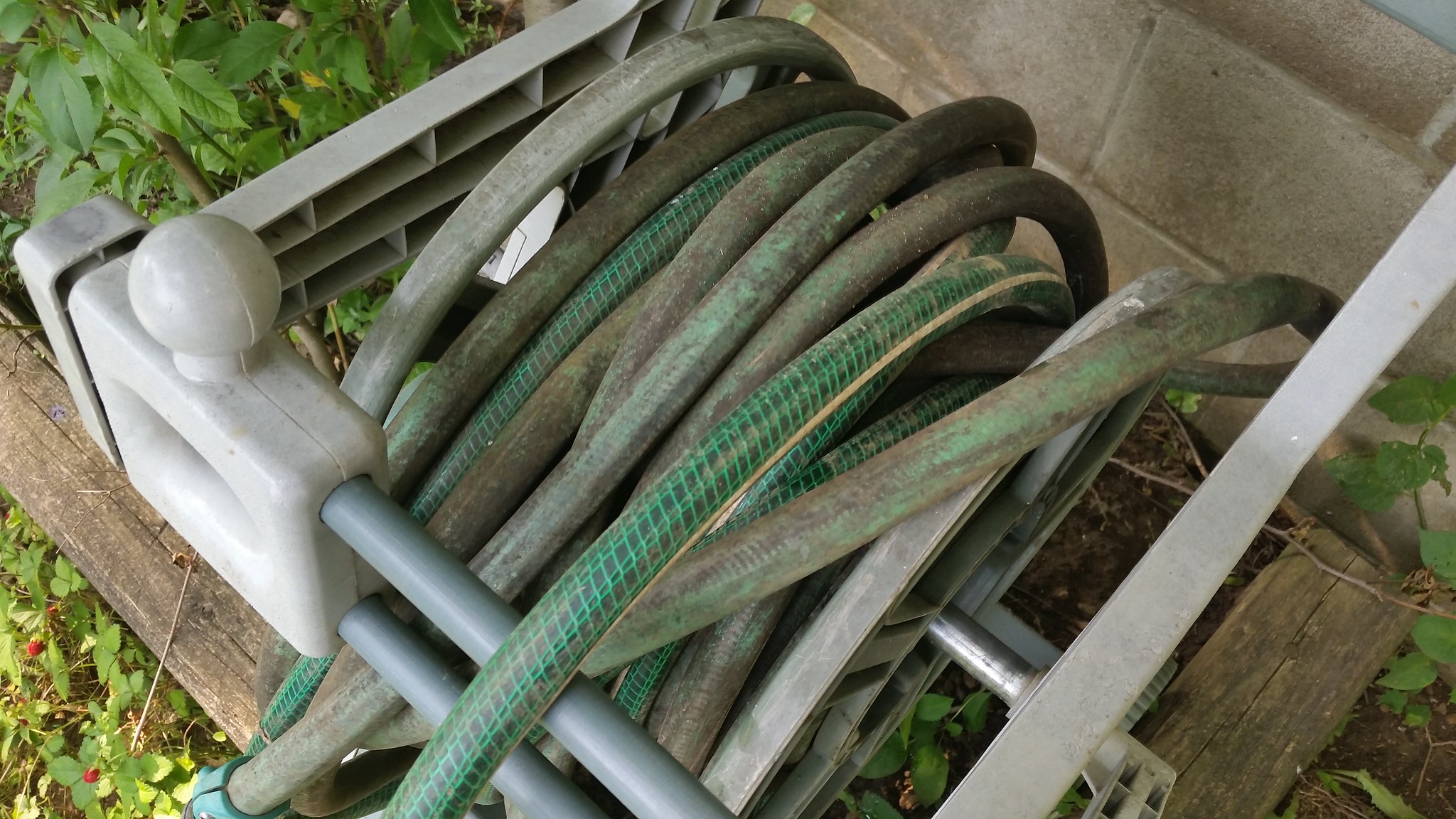This photograph captures a top-down view of a garden scene featuring an old, weathered garden hose coiled around a grey plastic hose reel. The hose, showing signs of age and wear, displays varying patterns and shades of green, from bright to matte, with sections visibly dirty and deteriorated. The plastic reel, with its slightly grimy appearance, consists of three larger parts and seems to be somewhat overwhelmed by the haphazardly wound hose, as parts stick out from the sides. To the left, a sizable lock secures the reel. The ground around the reel is a mix of dirt and decaying leaves, suggestive of a somewhat neglected garden bed dotted with plants, including wild strawberries and various green and brown foliage. In the background, a dirty white brick wall and some old wooden timbers frame the scene, enhancing the rustic, somewhat untended atmosphere of the garden area.